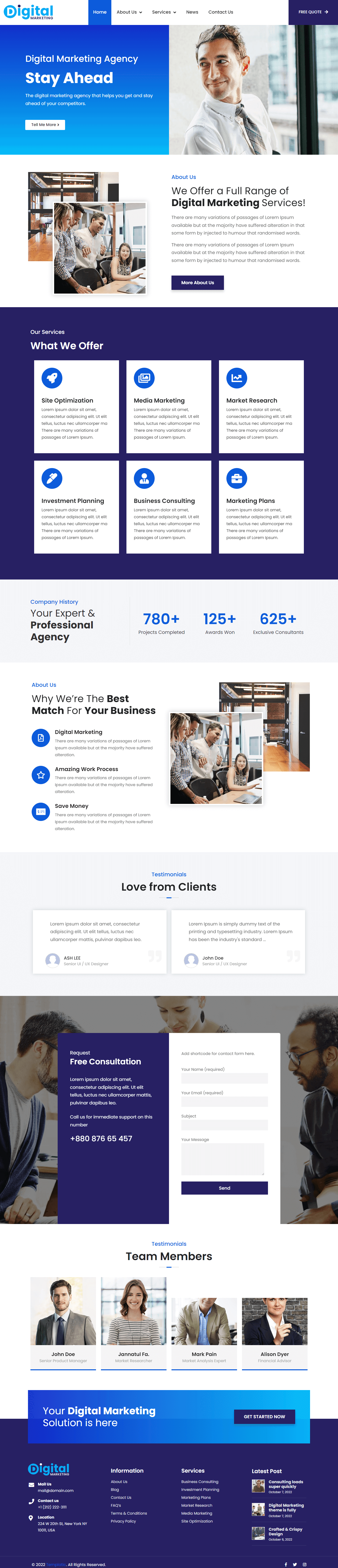This appears to be a slightly warped screenshot of a webpage belonging to a digital marketing agency, where the text is somewhat stretched, making small details hard to read. The resolution is low, but the main content remains discernible.

In the top left-hand corner, the text "Digital Marketing Digitalism" appears in blue. The navigation menu at the top reads "Home," "About Us," "Services," "News," and "Contact Us." The "Home" tab is highlighted in blue. On the right side, there’s a navy blue "Free Quote" button.

Below the navigation bar, the text "Digital Marketing Agency, Stay Ahead" is prominently displayed. An image of a man with brown hair, wearing a white dress shirt and gray tie, looking to the left, is featured beneath this text.

Further down, "About Us" is written, followed by the statement "We offer a full range of digital marketing services." Below this text is a blue "About Us" button. The section also contains two stock images depicting business activities.

Beneath these images is a navy blue box containing six white boxes, each with a blue icon or graphic. Accompanying text states, "Your Expert in Professional Agency," followed by three sets of statistics: "780+," "125+," and "625+."

The webpage continues with the header "Why We’re the Best Match for Your Business," displaying the previously seen stock images again. There are two client testimonials in white boxes.

Towards the bottom of the page, there is a navy blue box with the text "Request Free Consultation" and a provided phone number for contacting the agency.